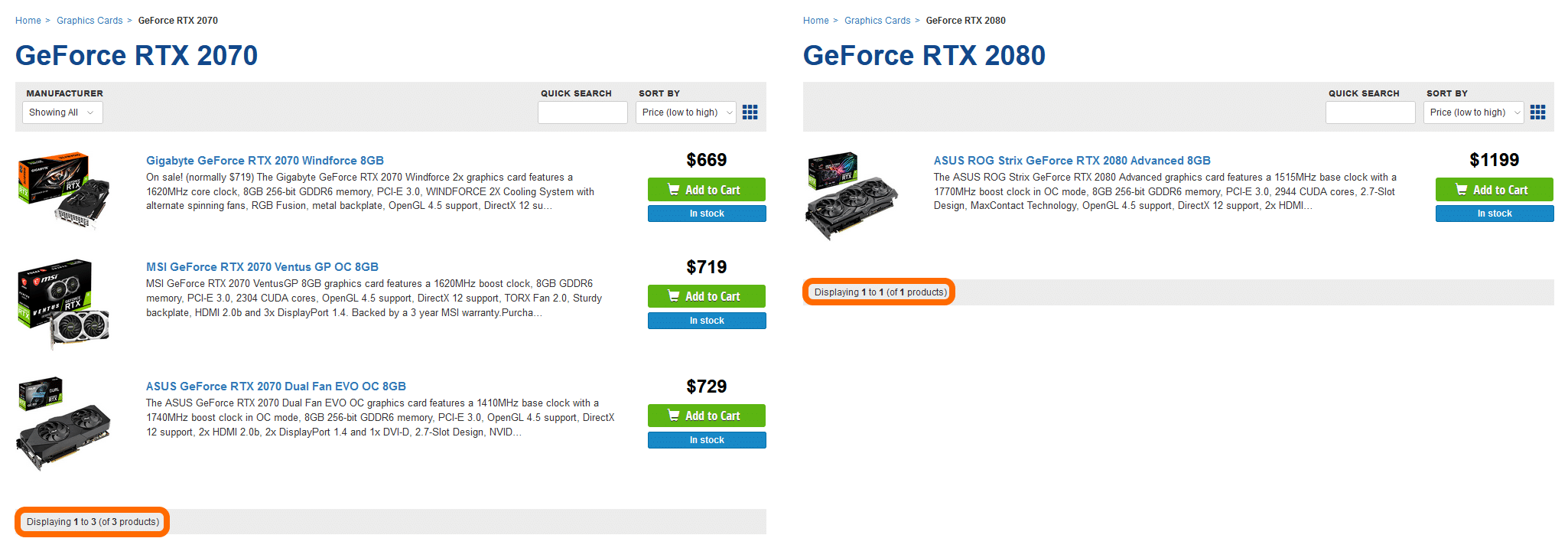This image is a composite screenshot of two separate desktop views of an online store webpage, focused on the sale of graphics cards. On the left side, it features three entries for the GeForce RTX 2070 graphics cards. The first entry presents a Gigabyte-branded card priced at $669, the second entry showcases an MSI card priced at $719, and the third entry lists an Asus card priced at $729. On the right side of the screenshot, there is a single entry for a high-end GeForce RTX 2080 card by Asus, specifically the ROG Strix model, which is listed at $1,199. Each entry includes an "Add to Cart" button alongside a smaller blue button that appears to indicate stock status, although the precise text is unclear due to its small and gray font.